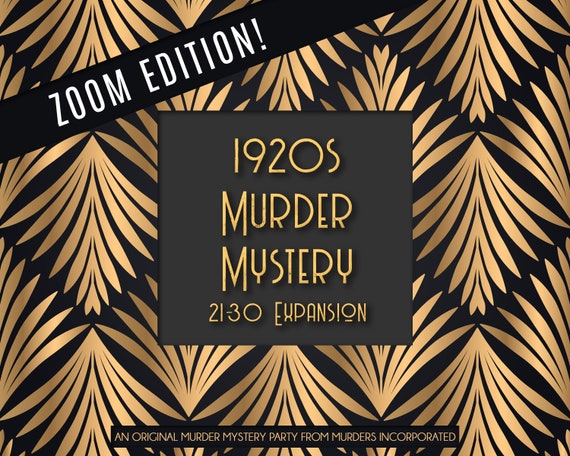This poster, likely originating from an online source, prominently advertises a Zoom Edition of a 1920s Murder Mystery 21-30 Expansion game. At the top left corner, a black diagonal banner displays "Zoom Edition!" in bold white capital letters. The central focus of the image features a gray square with "1920s Murder Mystery 21-30 Expansion" inscribed in gold letters, set against a black backdrop. At the bottom, a narrow black rectangle states "An Original Murder Mystery Party from Murders Incorporated" in white lettering. The background of the poster is decorated with an intricate pattern of golden bronze, beige, and tan leaves pointing both upwards and downwards. These leaves, varying in size and tapering at either end, create a dense, woven design against the black background, adding an elegant touch to the overall presentation.